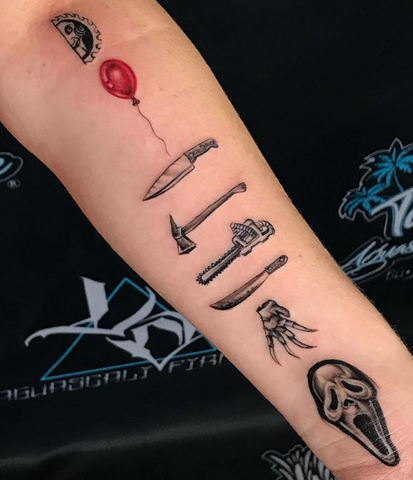The image is a vertically rectangular, full-color photograph, taken indoors under artificial light, clearly posed for. It features a close-up of a Caucasian person's arm, which extends diagonally from the top left corner to the bottom right corner. The background is a black banner or tarp with indistinct white and blue text, possibly forming shapes that vaguely resemble palm trees and a pyramid.

The arm is adorned with a series of detailed horror movie icon tattoos, starting from the elbow and moving down towards the wrist. At the top is a half-face of the clown villain, Jigsaw, from the Saw movie, partially merged with a saw blade. Below that is a red balloon, signifying the movie It. Next is a large butcher knife representing Michael Myers from Halloween. Following this is an axe, symbolizing The Shining. Further down is a chainsaw for the Texas Chainsaw Massacre, succeeded by a machete for Jason from Friday the 13th. The second last tattoo is of a clawed glove, iconic to Freddy Krueger from Nightmare on Elm Street. The last tattoo near the wrist is the ghost face mask of the killer from the Scream franchise.